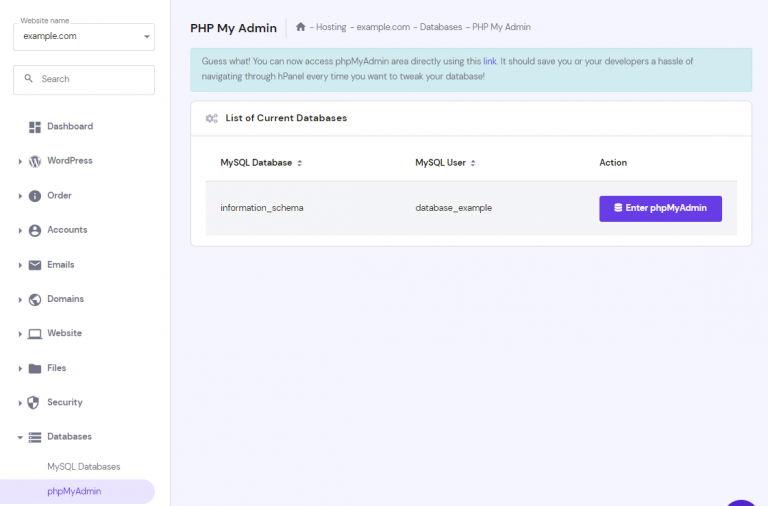Screenshot depicting a PHP My Admin interface, likely used for website development or management, divided into two main sections.

**Left Column (Navigation Pane):**
- **Background:** White with light gray accents.
- **Top Section:**
  - **Website Name:** "example.com" displayed in a drop-down menu within a light gray rectangle.
  - **Search Field:** Rectangular, featuring a magnifying glass icon and the word "Search."
- **Menu Items:** Listed vertically in gray, each with an icon:
  - Dashboard
  - WordPress
  - Order
  - Accounts
  - Emails
  - Domains
  - Website
  - Files
  - Security
  - Databases
- **Footer Text:**
  - Center-aligned text: "MySQL databases."
  - **Button:** "PHP My Admin" in purple letters on a lighter purple, rounded-oval background.

**Right Column (Main Content Area):**
- **Background:** Light purple with a blue tint.
- **Header:**
  - **Title:** "PHP My Admin" in large, bold, black letters.
  - To the right of the title, a vertical divider and a small house icon, followed by the path: "hosting-example.com-databases-phpmyadmin."
- **Informational Section:**
  - Rectangular box with text: "Guess what? You can now access PHP My Admin area directly using this link. It should save you or your developers the hassle of navigating through each panel every time you want to tweak your database."
- **Current Databases Section:**
  - **Title:** "List of current databases" 
  - **Table Headers:** "MySQL database," "MySQL user," and "Action."
  - **Database Entries:** Examples include "information_schema" and "database_example."
  - **Button:** "Enter PHP My Admin" under the "Action" column.

Overall, the screenshot provides a clear, organized interface for managing MySQL databases through PHP My Admin, with navigational and functional areas segregated for ease of use.